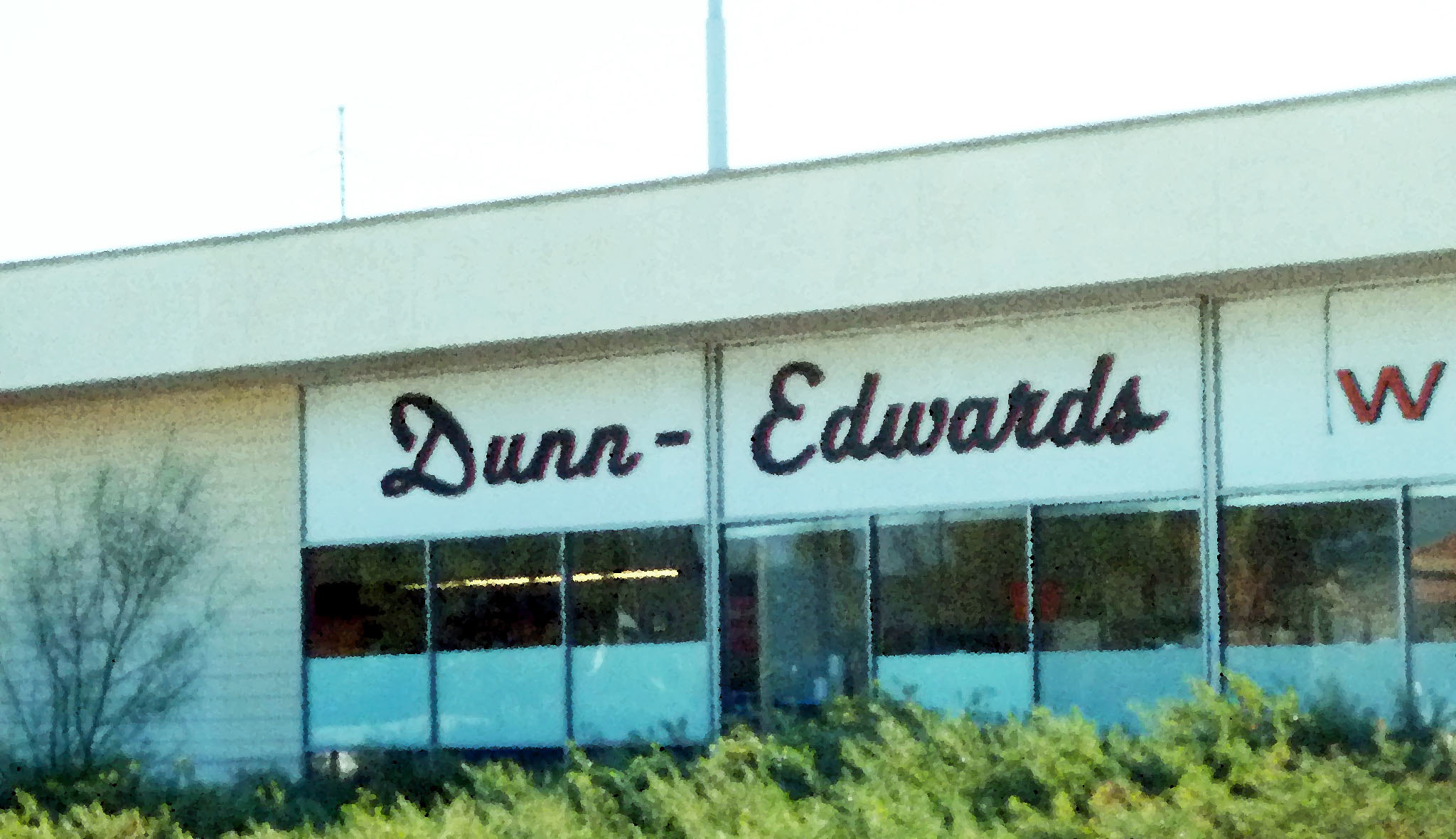The image depicts the exterior of a store named Dunn-Edwards. The store's name is prominently displayed in black cursive letters across the building's facade, with a red "W" adjacent to the logo. The store itself is predominantly white, although the left side features off-white siding. Through the large windows on the front of the building, some ceiling lights are visible, illuminating the indistinct items within. Below the windows, there is a white section that further accentuates the store's entrance.

In front of the building, a lush array of greenery, including bushes and grasses, adds a touch of nature to the scene. On the left side of the image, a tall tree stands prominently, enhancing the natural surroundings. Above, the sky appears bright and white, with a few poles extending upward, adding a subtle industrial element to the composition.